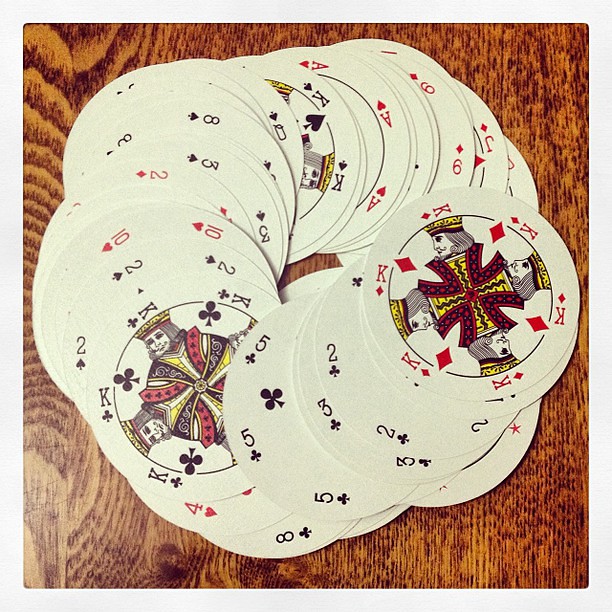The image depicts a unique deck of circular playing cards, arranged in a meticulous circle on a polished wooden surface. Prominently on the right side, the King of Diamonds is fully visible, accompanied by a mostly visible King of Clubs to its left. As the eye moves counterclockwise, the cards in view include the 2 of Clubs, 3 of Clubs, 5 of Clubs, and 8 of Clubs. Close by, the 4 of Hearts stands out. Continuing around the circle, the 2 of Spades, 10 of Hearts, 2 of Diamonds, 3 of Spades, and 8 of Spades come into view. Near the top, the Queen of Spades, King of Spades, and Ace of Hearts appear in sequence. Completing the circle, the 9 of Diamonds and Jack of Diamonds are also visible. The arrangement leaves a small circular space in the center, revealing the shiny, glossy texture of the wooden table underneath.